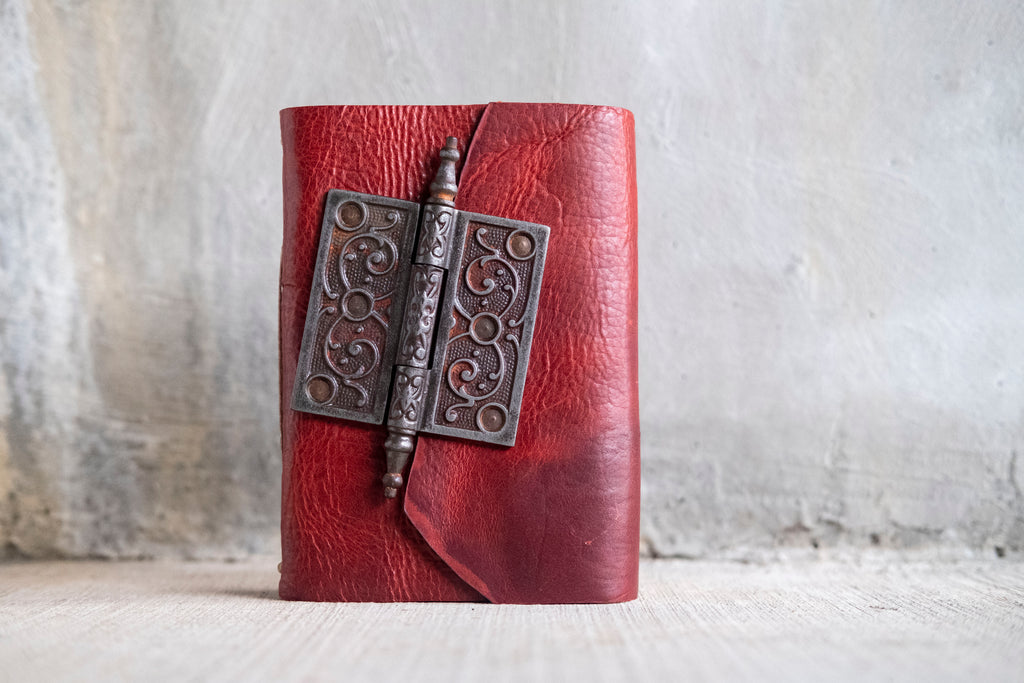This photograph depicts a vintage-style red leather artifact, possibly a wallet, journal, or satchel, standing upright against a rough, out-of-focus beige stucco wall and flooring. The leather cover is distressed and displays varying shades of brick red to reddish-brown. The centerpiece of the artifact is an ornate, antique door hinge-style clasp made of dark silver metal with elaborate engravings and filigree, featuring pointed and ornate ends. The hinge appears slightly askew, with a pin mechanism likely used to secure the cover closed. The weathered look of both the leather and metal, including a touch of rust on the hinge, complements the rough, textured background, giving the overall image a uniquely aged and handcrafted appearance.